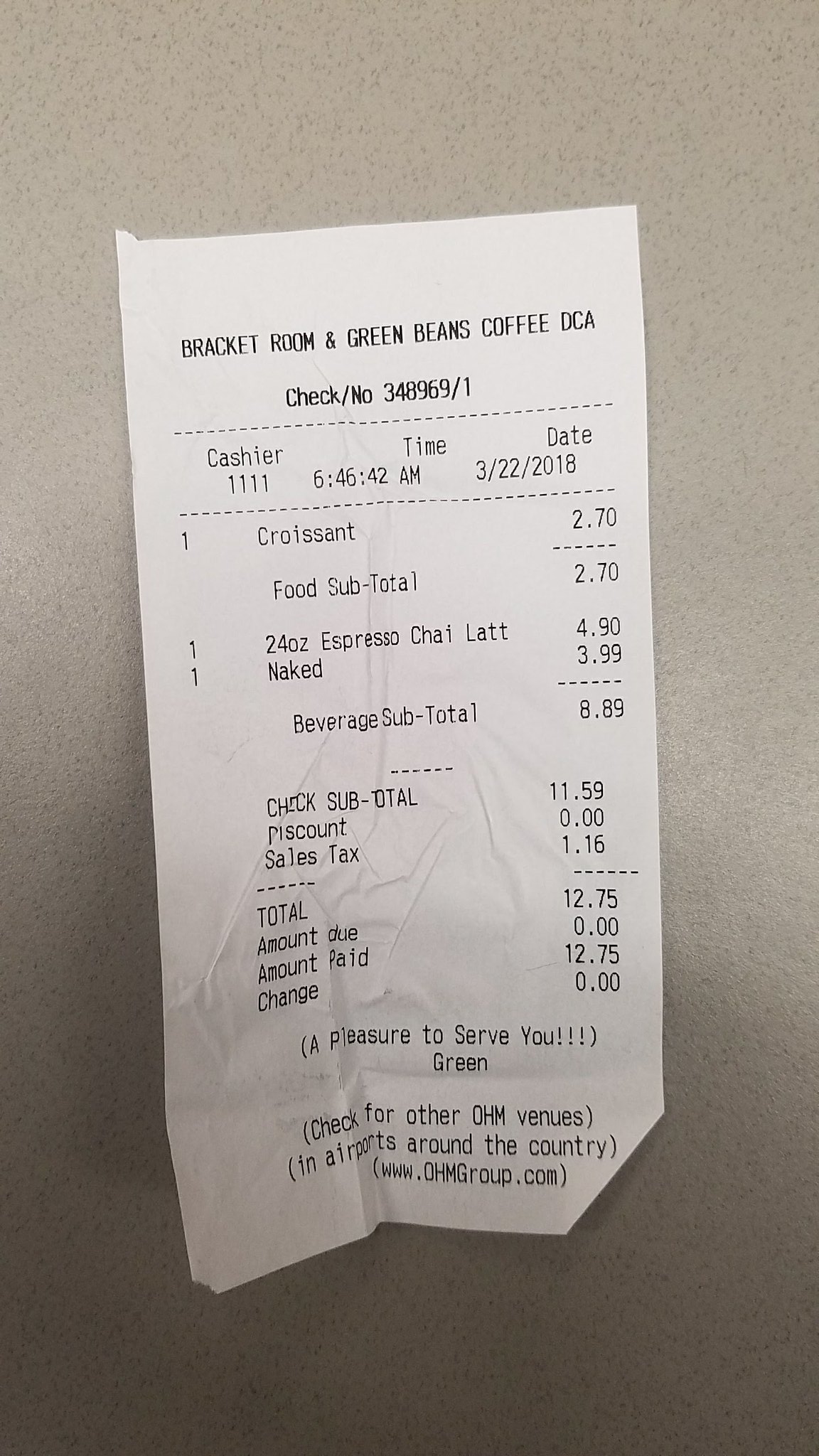The image displays a receipt placed on a white table. The receipt is white with black text and originates from Bracket Room and Green Beans Coffee at the DCA airport. The check number is 348969/1, handled by cashier 1111. The printed time is 6:46:42 AM on the date 03/22/2018.

The order includes:
- One croissant priced at $2.70.
- One 24-ounce espresso chai latte costing $4.90.
- One Naked beverage priced at $3.99.

The food total is $2.70 and the beverage total is $8.89, resulting in a check subtotal of $11.59. There were no discounts applied. The sales tax amounts to $1.16, bringing the total to $12.75. The amount due was zero as the full amount of $12.75 was paid, indicating no change returned. The receipt concludes with the message, "Pleasure to serve you," and encourages customers to check for other OHM venues at airports nationwide by visiting www.ohmgroup.com.